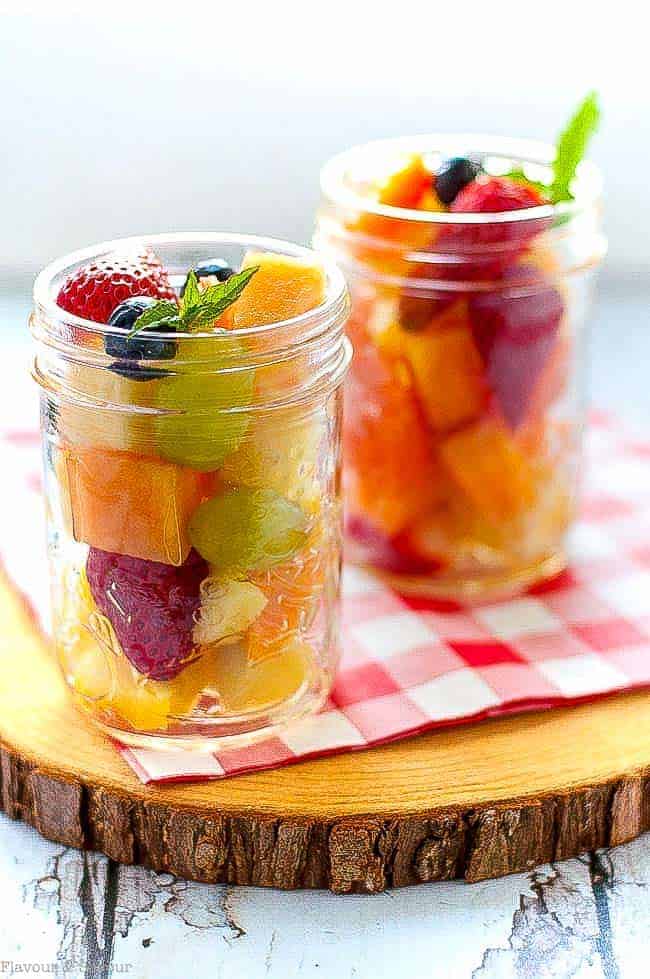In this vibrant photograph, we have two clear mason jars filled with an assortment of colorful fruits, arranged on a unique serving surface. The scene is set on a plate crafted from a sliced tree trunk, showcasing its golden-hued rings at the center and a dark brown, textured bark edge. The jars rest on a red and white checkerboard-patterned napkin. The jar on the left contains an enticing mixture of pineapple, strawberries, grapes, mango slices, and blueberries, with a sprig of mint adding a fresh touch. The jar on the right, slightly blurred in the background, features a colorful combination of orange, red, and yellow fruits. The entire setup is placed on a table with a gray wooden texture, and the overall image, free of people or text, evokes a rustic and appealing presentation, ideal for a recipe website.